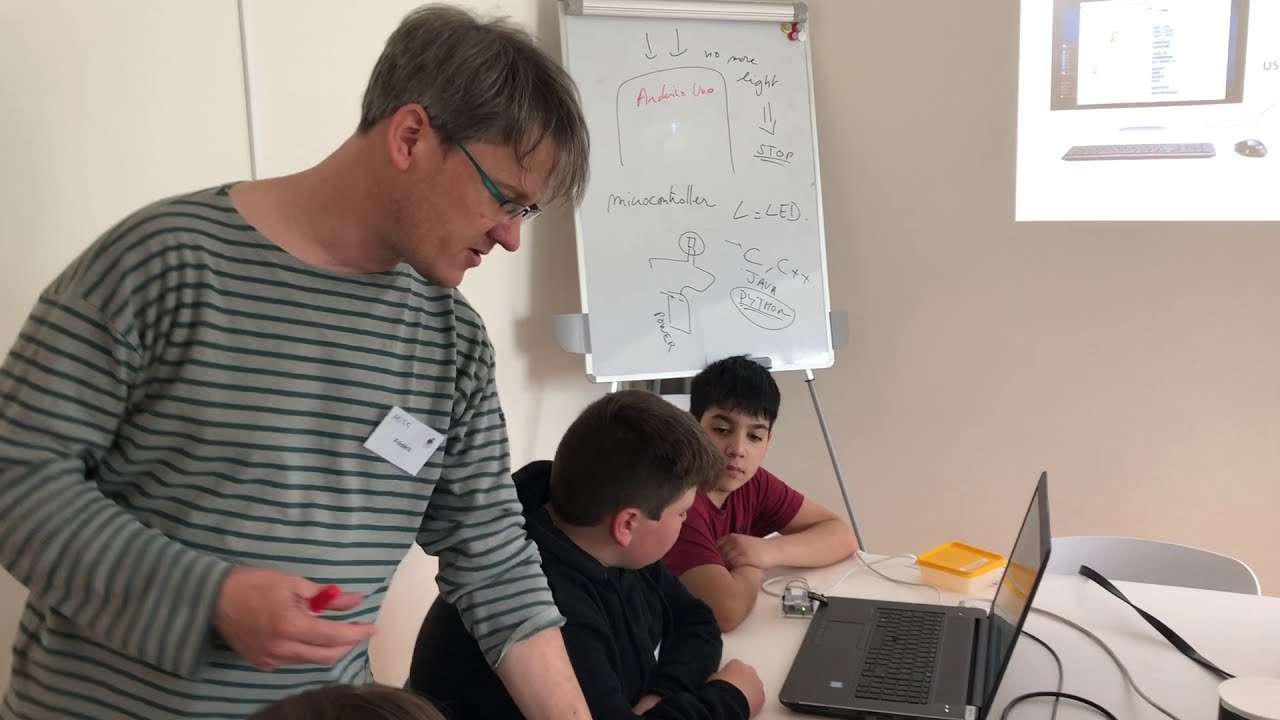In a well-lit classroom during the daytime, a teacher and two students are engaged in an activity around a white table. The teacher, a white male wearing minimal-rimmed glasses with blue arms and a long-sleeve gray shirt with black horizontal stripes, stands on the left side of the image. He holds a red-capped pen in his right hand and has a name tag pinned to his shirt, though the writing on it is illegible. 

Seated to his right are two boys. The first boy, sitting closest to the teacher, has short dark brown hair, a bit of redness on his cheeks, and wears a long-sleeve black shirt with his arms crossed in front of him. His fist is visible near an open black laptop on the table. The second boy, who appears to be of Hispanic descent, has black hair and wears a ribbon-colored, likely red, t-shirt. He looks down at the laptop screen, which is facing the first boy.

On the table, beside the laptop, there is a yellow-lidded plastic container, and various black wires are also visible. The background features a white drawing board filled with mostly black ink designs and some red ink lines, including arrows pointing down, an arch, and freehand words. In the upper-right corner of the image, light glares through a window with white framing. Beneath the table, the top of a chair is visible alongside the scattered wires. The classroom wall itself is white and plain, fitting the educational setting.